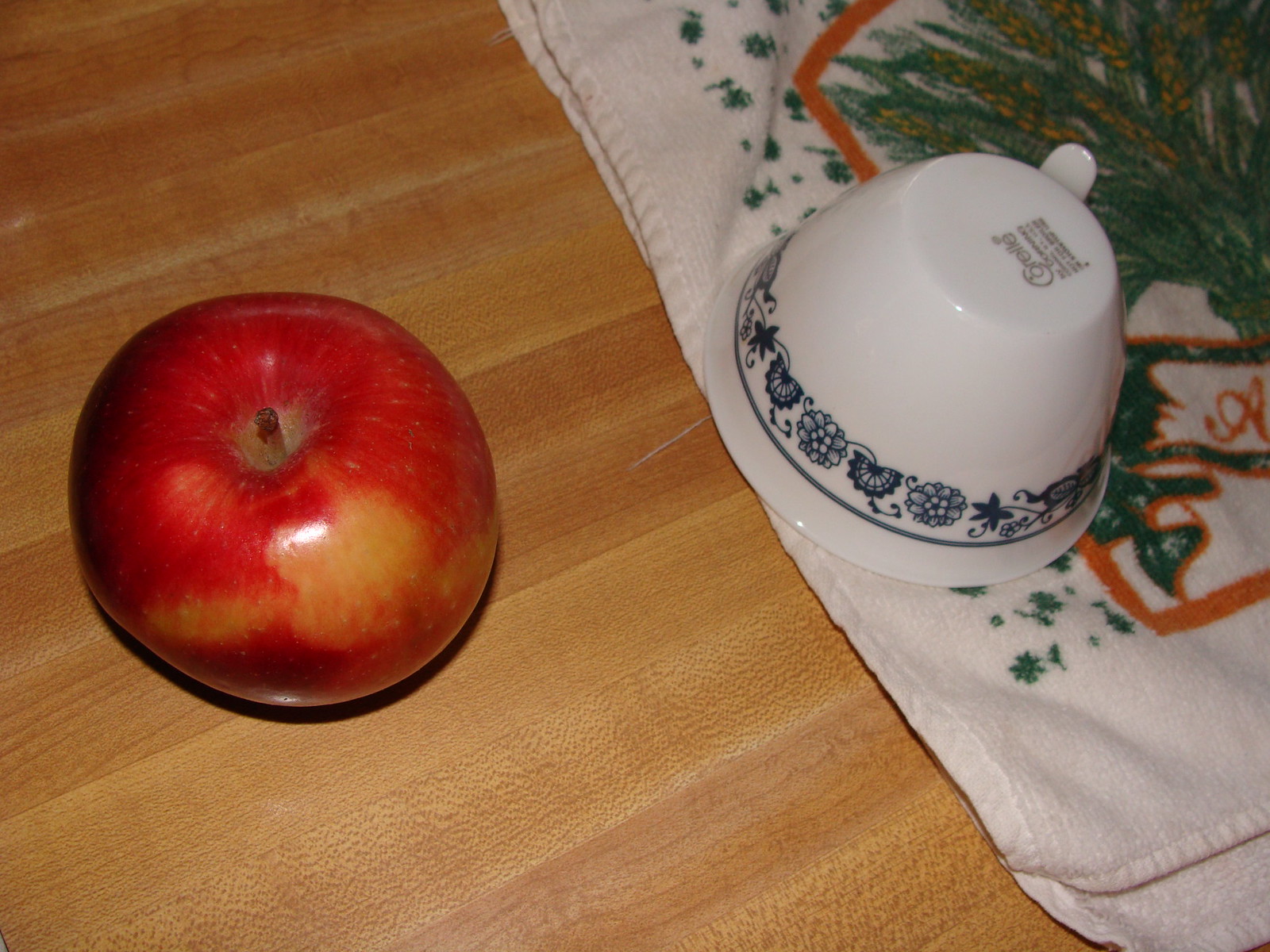This color photograph showcases a beautifully composed still life. On the left side, there is a medium brown hardwood table, exuding warmth and natural elegance. Atop the table sits a large, ripe apple with a glossy red skin streaked with hints of contrasting yellow, suggesting it might be a Fuji apple. The apple's vibrant colors and smooth texture catch the eye.

On the right side of the image, a cloth napkin adorned with intricate designs is neatly placed. The napkin features a pattern that closely resembles wheat stalks, depicted in green and yellow hues. It also boasts an orange border with delicate green embellishments beyond it, adding a touch of sophistication.

Additionally, a teacup is positioned upside down on the napkin. While the silver writing on the bottom of the teacup is not legible, its dark blue decorative rim provides a striking visual contrast. The teacup’s elegant design and the overall arrangement contribute to a harmonious and aesthetically pleasing scene.